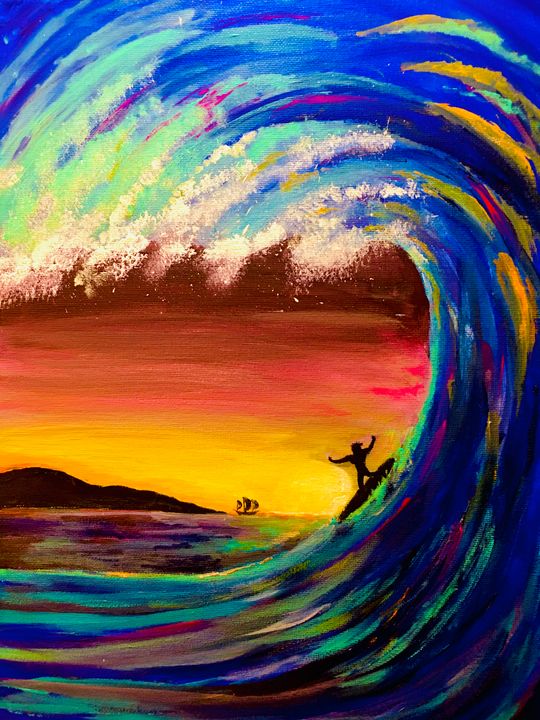This vertically aligned rectangular painting vividly depicts a scene of a person surfing a gigantic, colorful wave. The wave itself is an almost circular swirl starting from the lower left and curving up the right side, then looping back toward the left at the top. It is richly detailed with streaks of blues, reds, browns, greens, and yellows, highlighted by white tips that suggest the cresting motion of the water. In the midst of this dynamic wave, an outline of a person on a surfboard is visible. The surfer, extending their arms, appears lower center-right within the wave. The background features a dramatic blend of colors transitioning from yellow at the bottom, through red in the middle, to brown at the top, signifying a sunset. Additional details include a sailboat with three sails, more water, and the outline of land or mountains in the distance. The entire scene is encapsulated without any borders, enhancing the illusion of boundless energy and movement.